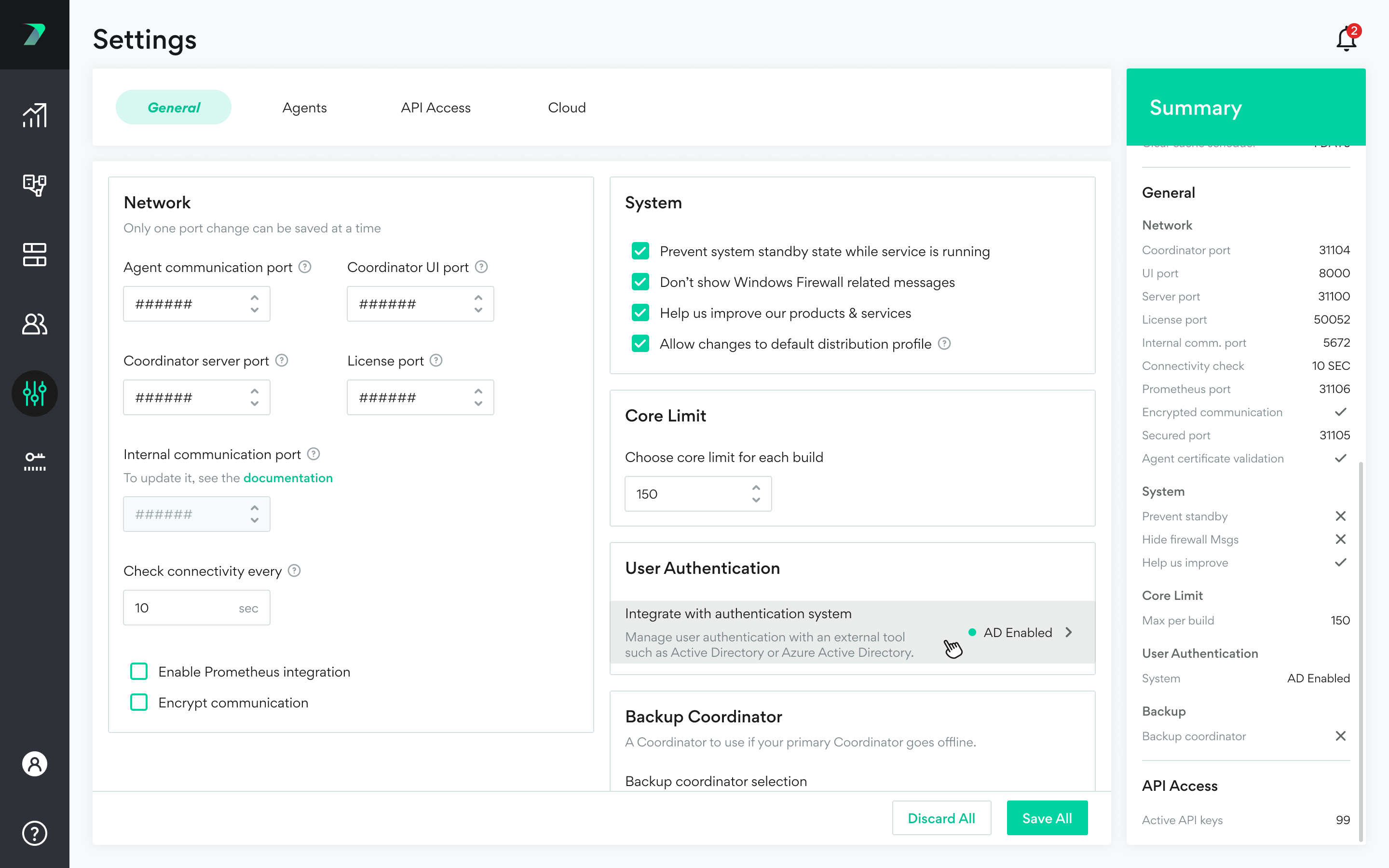**Image Caption:**

The image showcases a web application's settings page, prominently displayed on a white background. In the top left corner, the word "Settings" is written, indicating the section of the app being viewed. Below the settings header, there are four tabs—General, Agent, API Access, and Cloud. These tabs are colored black, except for the "General" tab, which is selected and highlighted in green.

The page contains various sections and fields for configuration:

- **Network Section:** 
  - Includes a note stating, "Only one port change can be saved at a time."
  - Contains text fields or drop-down menus for input.

- **Agent Communication:**
  - **Coordinator UI Part**
  - **Lessons Part**
  - **Coordinator Server Part**
  - Below this, it states, "Internal communication part to update it, see the documentation."

- **Connectivity Check:**
  - Indicates, "Check connection connected with every 10 seconds."

- **Integration Options:**
  - Two unchecked checkboxes for enabling Prometheus integration and crypt communication.

On the right side, the top header reads "System," featuring four checked options indicated by green ticks:
  - Prevent system standby state while the service is running.
  - Don’t show Windows Firewall related messages.
  - Help us improve our products and services.
  - Allow changes to the default distribution profile.

Additional options include:
  - **Column settings** for each build, set to 150.
  - **Authentication options:** Use authentication and integrate with the authentication system (AD enable).
  - **Backup Coordinator:** A section dedicated to backup settings.

The top-right corner features another green-highlighted section labeled "Summary," summarizing various configuration and system settings, including Network, Coordinator, UI, Server, License, Internet.com.port connectivity check, Prometheus, Encrypted communication, Secured port, Agent certification, validation, and System settings.

At the bottom of the page, there is a section for API Access, followed by two buttons: "Save All" (highlighted in green) and "Discard All," facilitating user actions to save or discard the changes made.